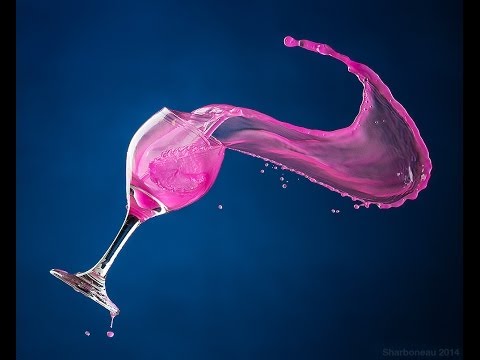The image is a dramatic and vibrant commercial photograph featuring a medium-sized clear glass wine goblet in the midst of dynamic motion against a deep blue to black gradient background. The goblet, tilted to the right, contains a striking bubblegum pink liquid, which is captured in a stop-action effect as it swirls out of the glass in a dramatic U-shaped wave. This pink liquid forms a large, flowing arc with scattered droplets trailing above and near the stem of the glass, creating the illusion of motion and energy. Despite the liquid’s vigorous splash, the goblet remains three-quarters full, which amplifies the visual impact. The contrast between the rich, dark background and the vibrant pink liquid, along with the precise, manipulated photography technique, suggests the image could be an artistic advertisement. The photograph’s dimensions are approximately 10 inches wide by 8 inches tall, adding to its substantial and impactful presence.